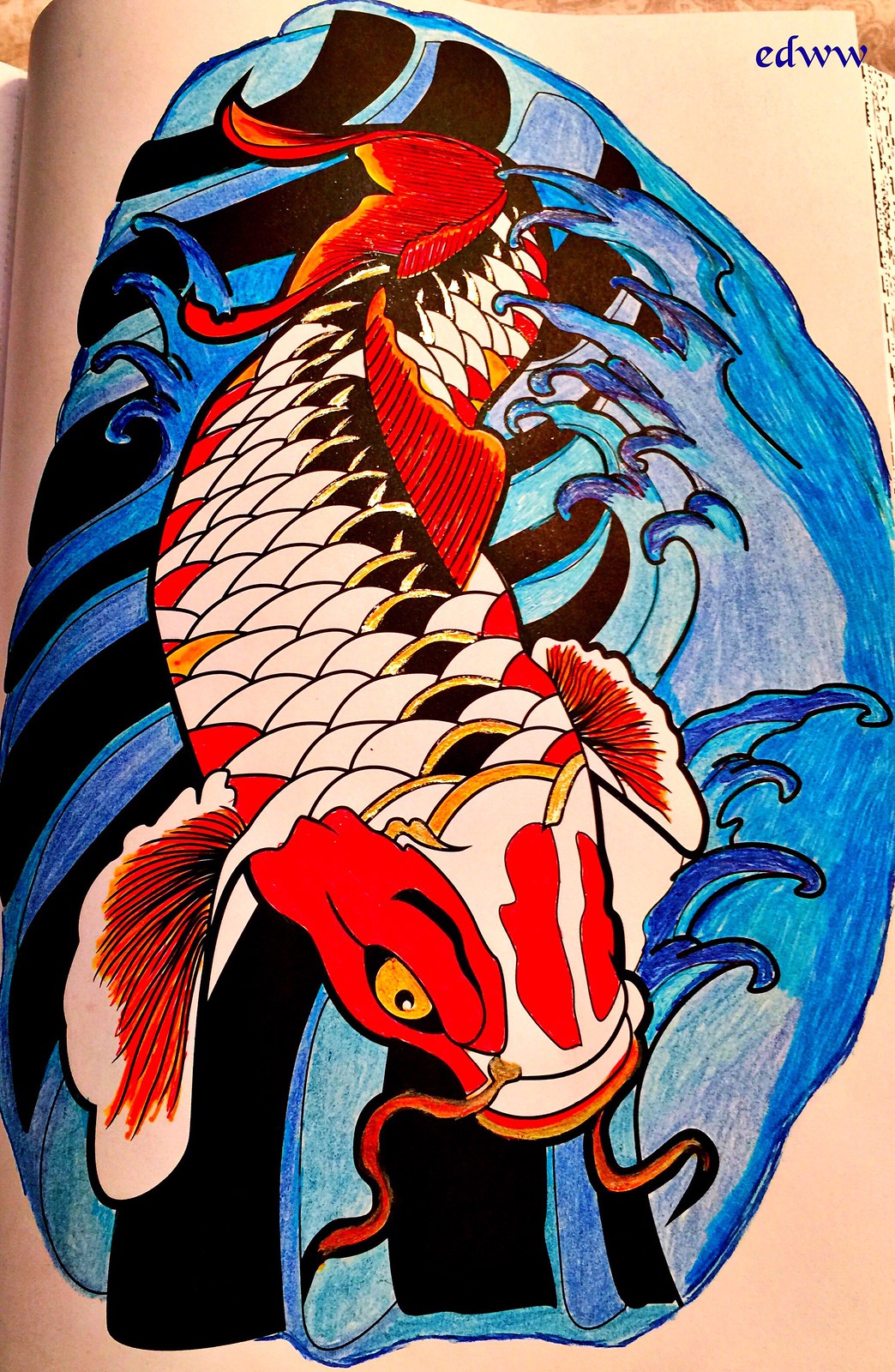This imaginative painting depicts a whimsical fish characterized by its vibrant colors and distinct features. Dominating the composition, the fish is primarily red and white, with a striking yellow circle and a central black dot adorning its frontal section. Extending gracefully from this focal point are two delicate, red, wispy whiskers that add a touch of elegance to the creature.

The fish is submerged in dynamic blue waters, where expressive waves imbued with black shadows swirl around it, enhancing the sense of movement. Running lengthwise down the middle of the fish, a bold black and gold stripe provides a striking contrast against the otherwise predominantly white body. Accentuating the composition are a couple of red markings on either side of the fish, complementing its vibrant palette.

Crowning the fish, the top-most part boasts a deep red hue intertwined with intricate black lines, adding depth and texture to the overall appearance. The detailed artistry unmistakably conveys the essence of a fish, further confirmed by the inscription "EDWW" in the top right corner of the painting, adding a playful touch to the captivating scene.